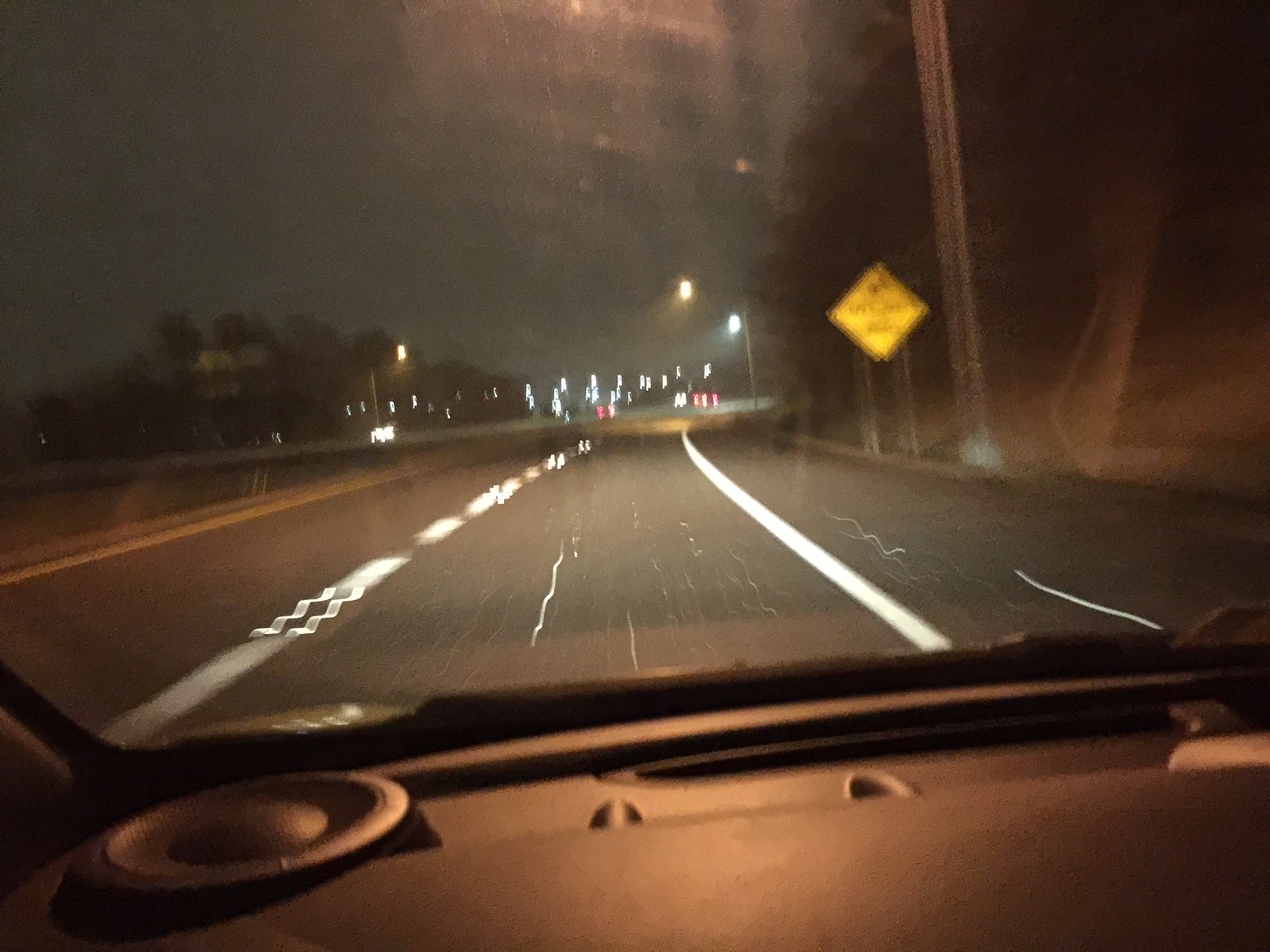A blurry nighttime photo taken from inside a car, likely by a passenger, captures a scene of a multi-lane road. The black dashboard of the car is visible at the bottom of the image. The road, which has at least four lanes, is divided by a barrier with two lanes heading in the photographer’s direction and two lanes for oncoming traffic. The road features white and yellow painted lines, indicating lane boundaries. Multiple cars are seen ahead, their taillights glowing red, while headlights from oncoming traffic shine toward the camera. Streetlights are intermittently visible along the road, with one shining directly onto the car's windshield. There are also blurry signs visible to the right and left, although their text is unreadable. Flanking the road are trees, delineating the perimeter without any buildings in sight. The night sky appears gray, devoid of any celestial objects.